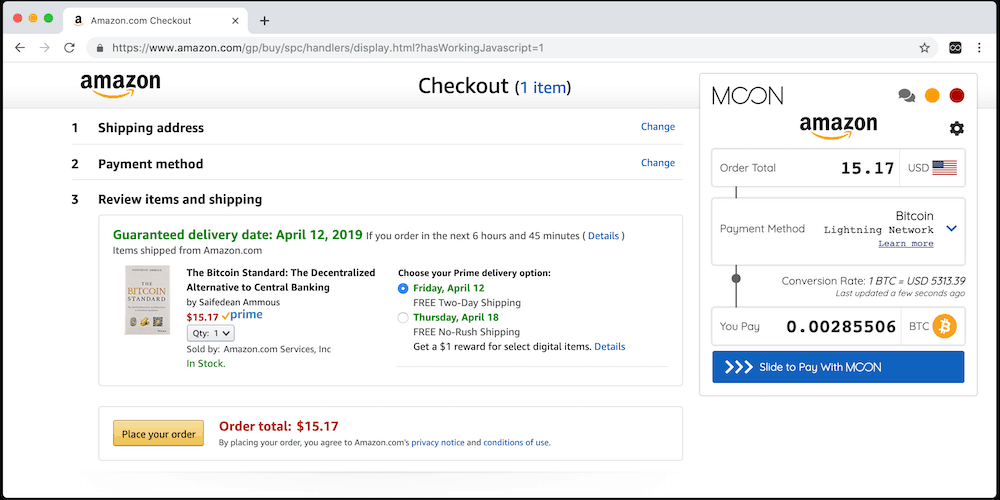This screenshot captures the checkout page on Amazon.com. At the top left corner of the browser, the traffic light colors (a horizontal arrangement from left to right) feature a red dot, a yellow dot, and a green dot. Next to these dots is the Amazon tab.

In the main view of the screenshot, the Amazon logo is prominently displayed, with "Amazon" written in black text and a yellow arched arrow underneath the letters "M" "A" and "Z."

The user has selected to purchase the book titled "The Bitcoin Standard: The Decentralized Alternative to Central Banking." The book is priced at $15.17 USD, and an option to pay with Bitcoin is available, with the equivalent amount being 0.00285506 Bitcoins. 

The user has opted for Prime delivery, which offers free two-day shipping, with the expected arrival date being Friday, April 12th. The order has not yet been finalized, as indicated by the yellow "Place your order" button located at the bottom of the page.